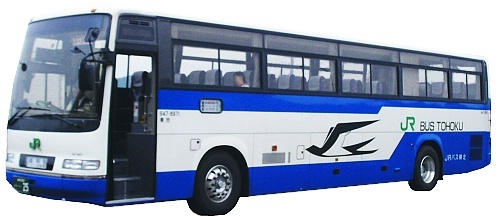This image features a blue and white city metro bus set against a plain white background. The bus, approximately 15 to 20 yards long and 6 to 7 feet wide, has a very flat front with a large, flat windshield. The doors are positioned on the left side of the bus, revealing steps leading into the interior, where gray seats are visible. One passenger is seated inside near the front. The bus displays a black and white bird logo, resembling an origami bird in flight, on its side. The lettering "JR" appears in green on the front of the bus, while "Bus to TOHOKU" is written at the back, accompanied by another logo. The headlights are off, and the license plate is not visible.